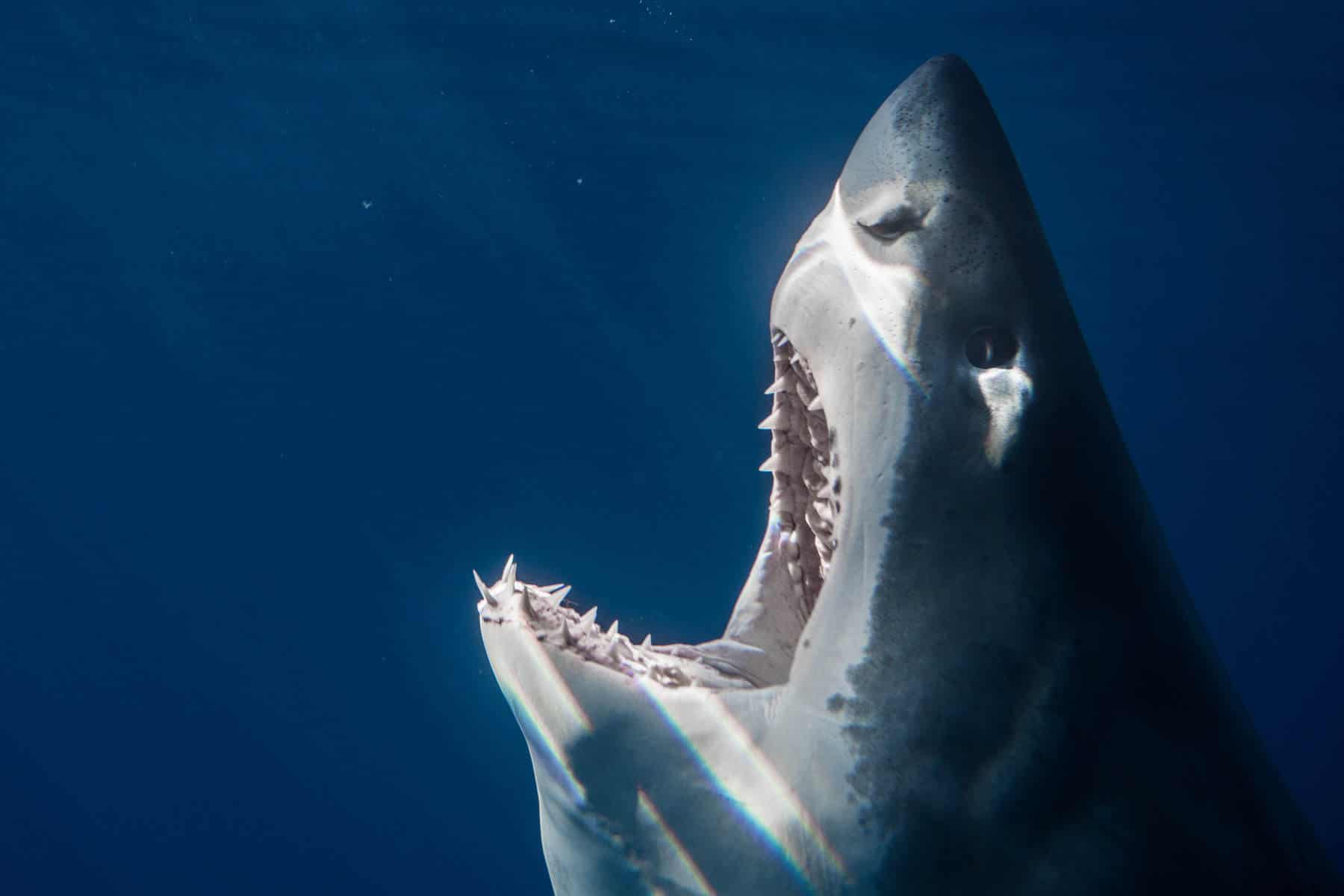The underwater scene captures a dramatic image of a formidable great white shark with its mouth gaping wide open, revealing stark white, jagged teeth. The shark is oriented upwards, its nose nearly touching the top of the frame. The background is a dark blue ocean, interspersed with streaks of light filtering down from above, creating a striking contrast against the deep water, which adds texture resembling starry dots.

The shark dominates the composition, and the right side of its body and face are clearly visible. The creature’s gray-toned head transitions from darker hues at the top to lighter blues along the lower half of its face. A notable feature is the pinkish-purplish interior of its aggressive gape. 

Prominent details include a light streak across its sinister black eye and a curved white mark behind it. An intricate horizontal slit accentuates its nose, highlighting its nostrils. As light penetrates the water, some areas near its open mouth appear lighter blue, enhancing the dramatic effect. The imposing image underscores the awe-inspiring, yet menacing, presence of the great white shark in its natural ocean habitat.